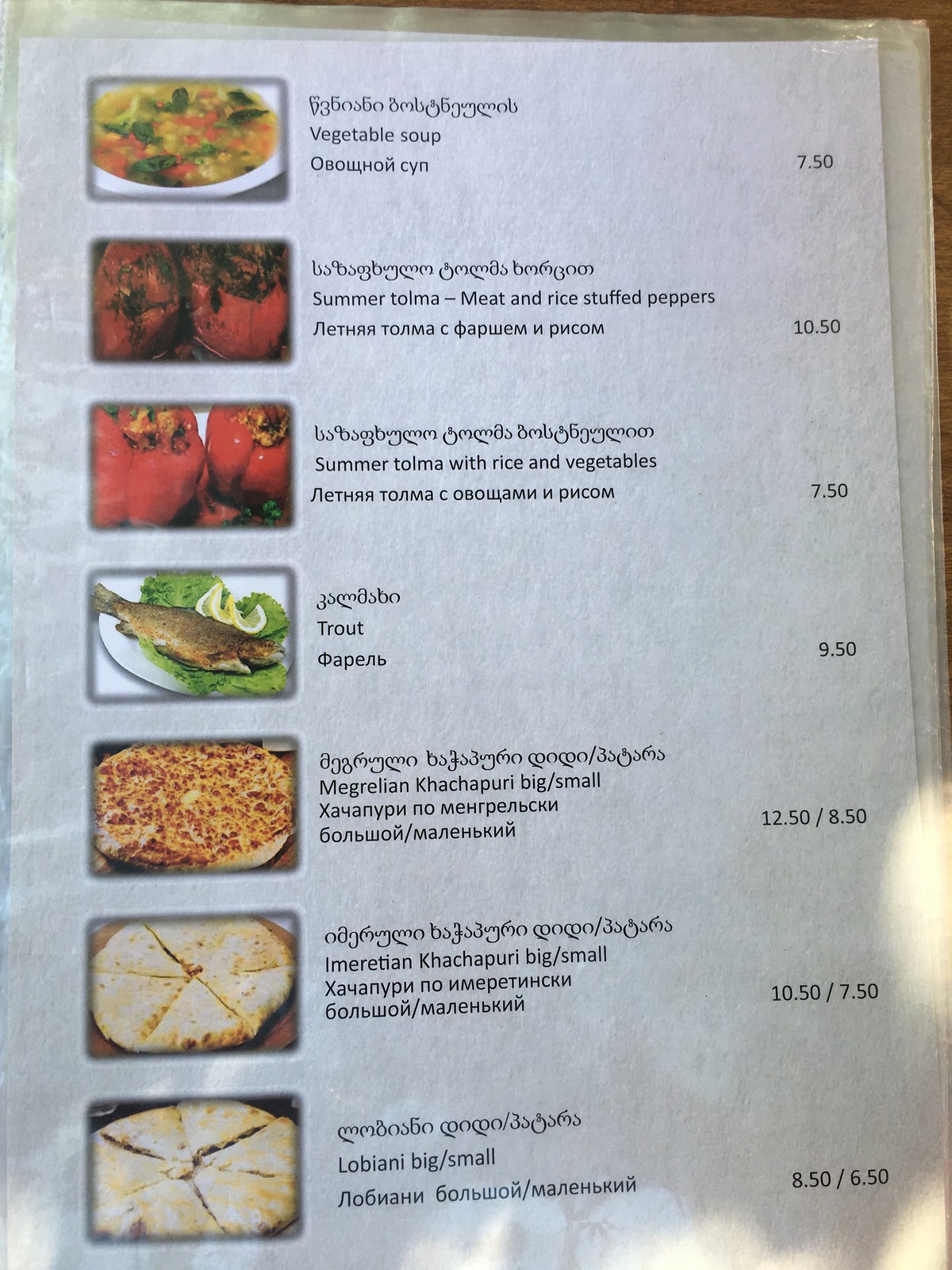This photo captures an intricately detailed menu, printed on textured paper, displaying a diverse selection of seven items. The menu layout features each item depicted within individual rectangular boxes situated on the left-hand side, providing a visual representation for clarity. Adjacent to these images on the right-hand side are corresponding price tags, clearly marking the cost of each dish.

The offerings include:
1. Vegetable Soup
2. Summer Tomato with Rice and Vegetables
3. Trout
4. Melgarine
5. Capuchin

Additionally, the menu lists options in varying sizes such as "Big" and "Small," along with several other items that are challenging to pronounce.

The text on the menu is bilingual, with Russian script positioned below each item and an elaborate Armenian script set above, adding to the authenticity and cultural richness of the menu. This juxtaposition of languages provides a glimpse into the diverse culinary traditions represented.